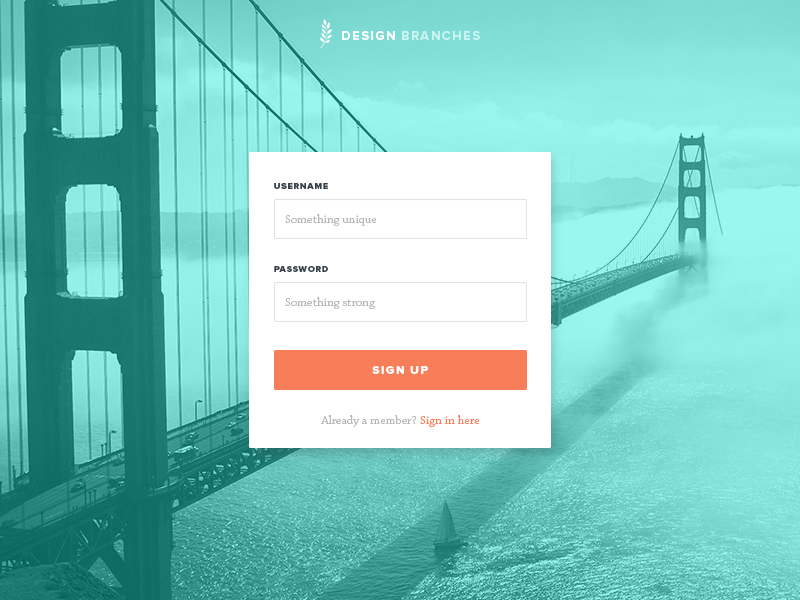In this image, a long bridge spans across the background with several vehicles traveling along it. In the center of the image, a digital interface captures attention, featuring a username field and a password field. The username field is notable for its unique entry, while the password field indicates a strong password. Below these fields, options for 'Sign Up' and 'Already a member? Sign in here' are prominently displayed. The interface also includes a 'Close your R' button, highlighted in blue, white, and orange. At the top of the image, decorative design elements resembling branches add an artistic touch.